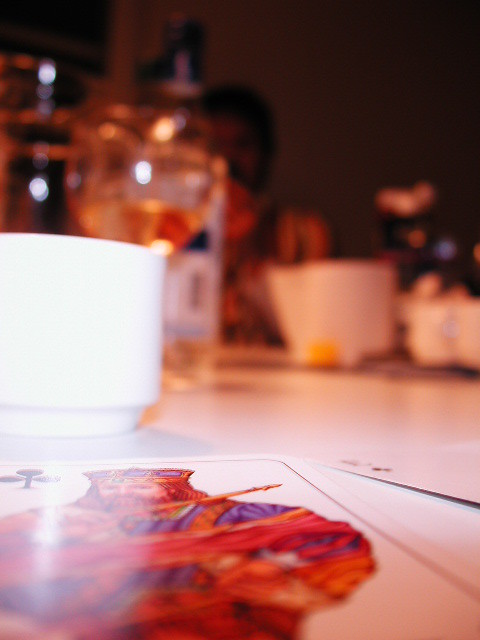A close-up image captures an intense moment in a card game. Dominating the foreground is a zoomed-in view of the King of Clubs card, showcasing the king's ornate attire and hat, although the 'K' is partially cut off. Right beside it on the table lies an Ace of Clubs. Adjacent to these cards, a white cup is prominently placed, and shiny clear bottles glisten in the light toward the left-hand corner. On the opposite side, another cup that resembles the first one is visible. Furthermore, there's a ceramic item on the right with a blue dot and two rose-colored dots, likely reflections. The background appears blurry, especially in the upper left corner, where shadows from the objects cast by the lighting add depth to the scene. A person is dimly visible in the far back, obscured by the array of cups and bottles, adding a mysterious element to the ambiance.